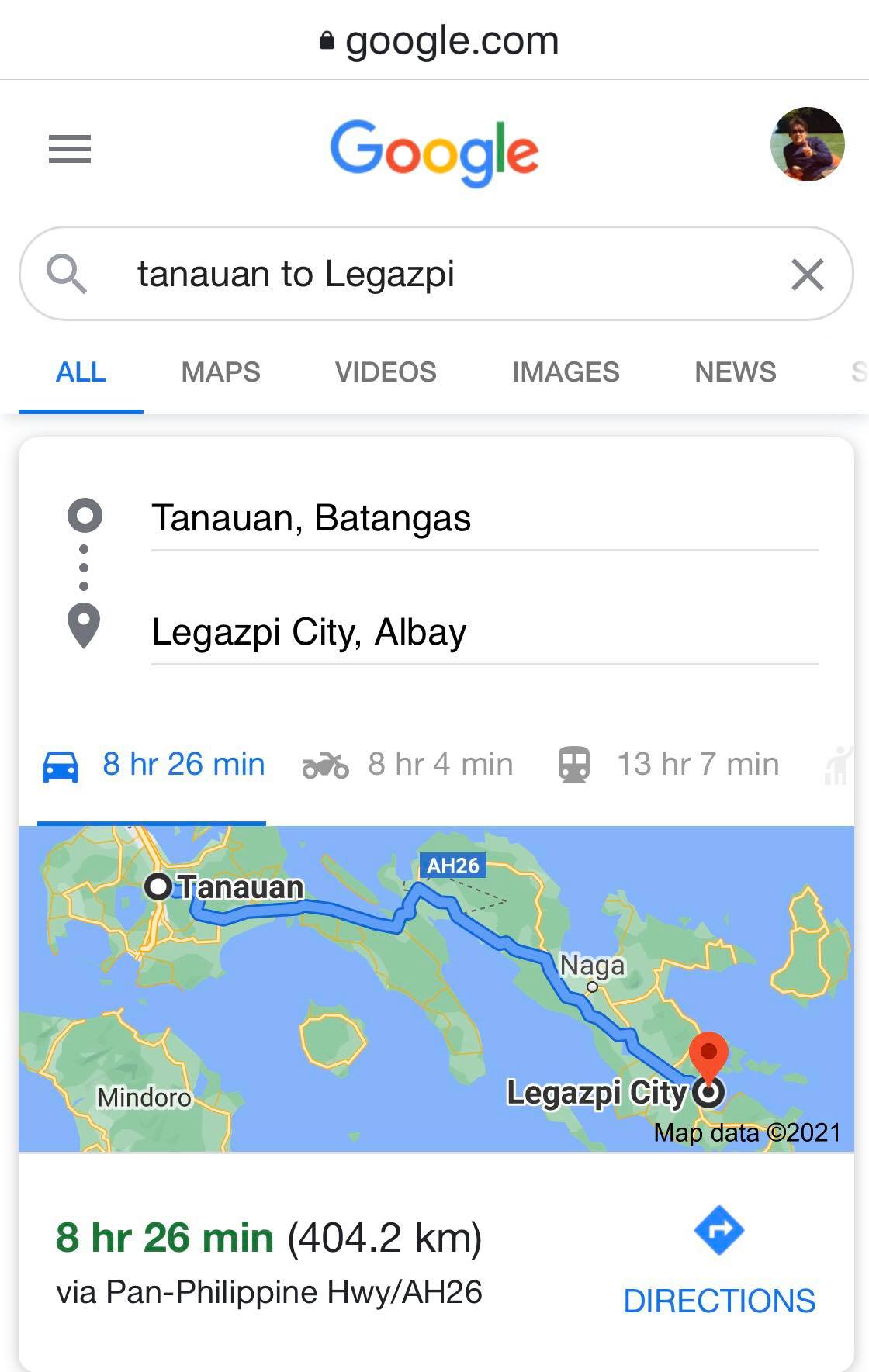This is a detailed screenshot of a Google search page on the Google.com domain. At the top center of the screen, "Google.com" is displayed with a secure lock symbol beside it, indicating a secure connection. The user is logged into their Google account, as evidenced by a profile picture of a woman wearing sunglasses in an outdoor setting, located in the upper right-hand corner of the screen. 

In the central search bar, the text "TANAUAN to LEGAZPI" is entered. Below the search bar, the search filter options—All, Maps, Videos, Images, and News—are displayed, with "All" selected and highlighted in blue with an underlined blue bar for emphasis.

Further down, the search results show directions for the queried route from Tanauan to Legazpi. The results provide estimated travel times for different modes of transportation: 8 hours and 26 minutes by car, 8 hours and 4 minutes by motorcycle, and 13 hours and 7 minutes by bus.